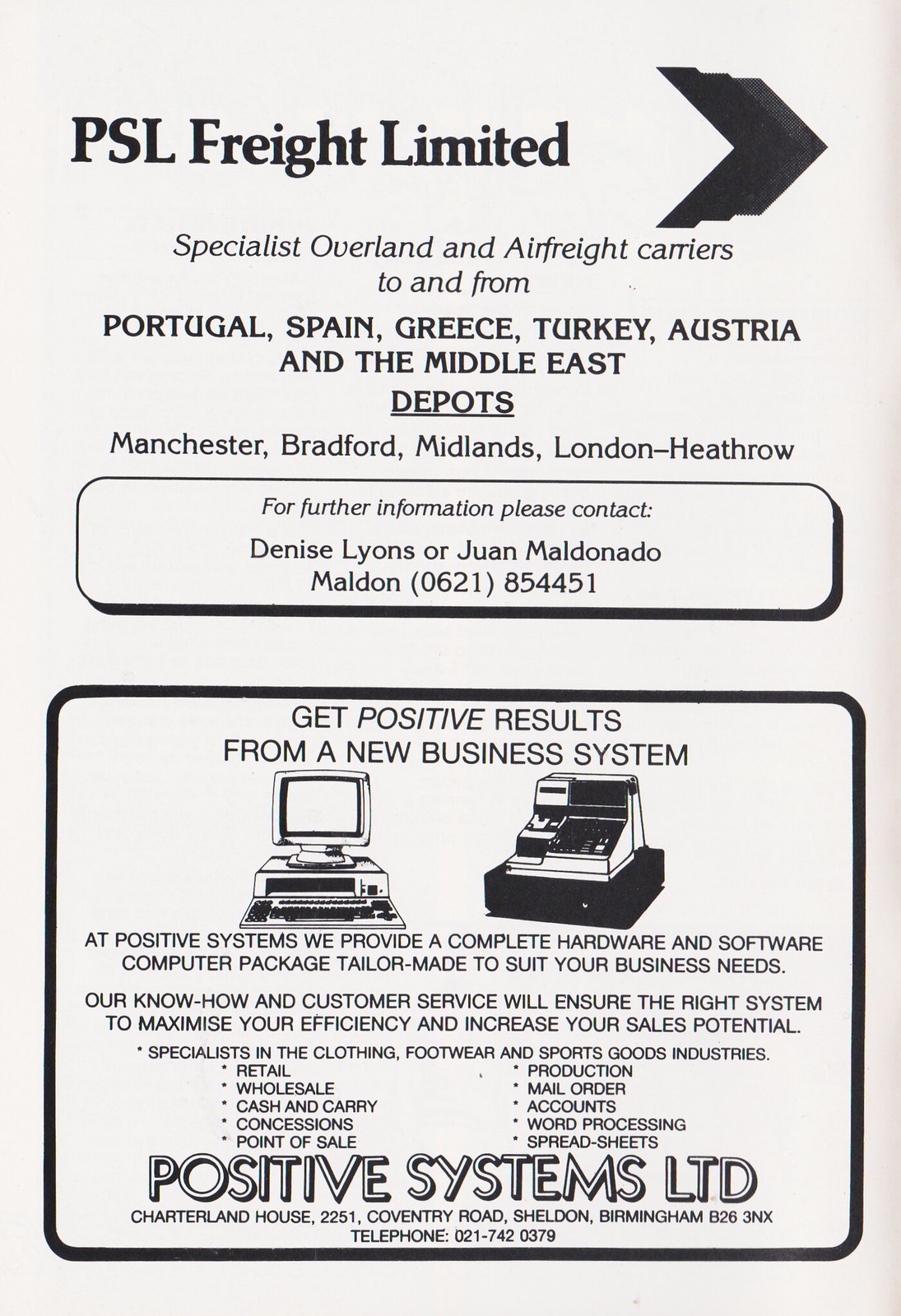This image is a vertically aligned rectangular business poster on white paper with black ink. At the top, in bold black letters, it reads "PSL Freight Limited." Below this, it announces "Specialist Overland and Air Freight Carriers to and from Portugal, Spain, Greece, Turkey, Austria, and the Middle East." The word "Depots" is underlined, followed by the locations: Manchester, Bradford, Midlands, London, Heathrow. A rounded rectangle below this contains contact information, stating, "For further information please contact Denise Lyons or Juan Maldonado Maldon (0621) 854451."

In the bottom half of the poster, another rounded rectangle includes the text "Get Positive Results from a New Business System." It features images of a computer and keyboard on the left and a cash register on the right. The accompanying text promotes, "At Positive Systems, we provide a complete hardware and software computer package tailor-made to suit your business needs. Our know-how and customer service will ensure the right system to maximize your efficiency and increase your sales potential. Specialist in the clothing, footwear, and sports goods industries: Retail, wholesale, cash-and-carry, concessions, point-of-sale, production, mail orders, accountants, word processing, and spreadsheets." At the bottom, in large bold letters, it says "Positive Systems LTD," followed by the address "Charlotte Land House, 2251 Coventry Road, Sheldon, Birmingham B26 39X," and contact number "021-742-0379."